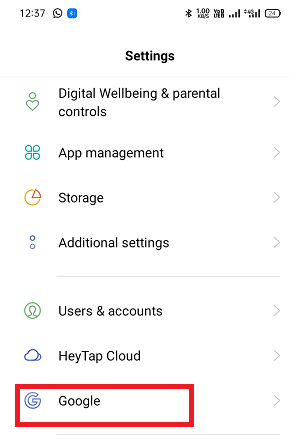A screenshot of the "Settings" section on a mobile phone display. Located at the top left corner of the screen, the "Notifications" headline shows "1237" accompanied by a speech bubble icon and a Bluetooth icon. On the top right corner, a battery icon indicates 24% charge, alongside icons for data speed (1 kb per second) and cellular signal bars.

At the center of the screen, the word "Settings" is prominently displayed, with a list of seven items below it. Each item is organized in a row featuring both an icon and a descriptive name:

1. **Digital Well-being & Parental Controls** - Represented by a green heart with a circle above it.
2. **App Management** - The icon details for this item are not specified.
3. **Storage** - Illustrated by a pie chart icon.
4. **Additional Settings** - The icon details for this item are not specified.
5. **User & Account** - Depicted by a green silhouette icon.
6. **HeyTap Cloud** - Represented by a cloud icon.
7. **Google** - Marked with a boxed-in red Google "G" icon, where the "G" is blue.

Each row contains an arrow pointing to the right, indicating that tapping the row will navigate to additional settings or options.